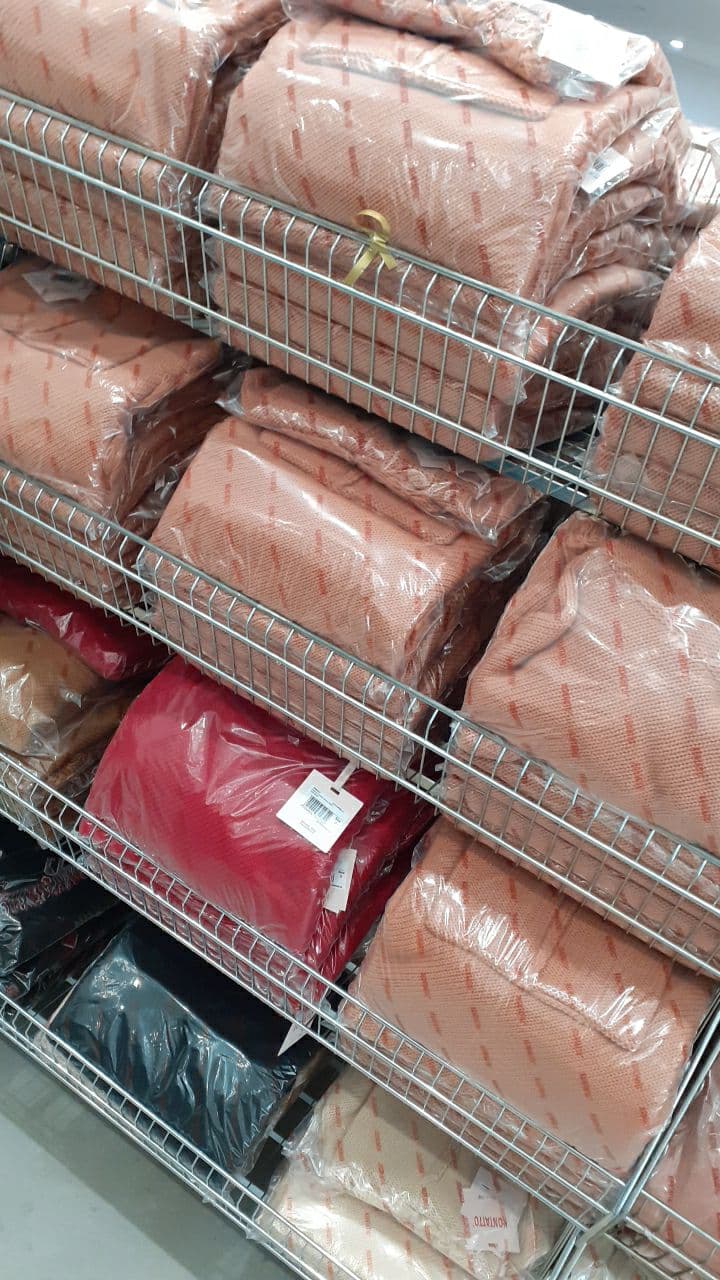The photograph showcases a metal rack with four rows of shelving, each containing three bales of clothing materials neatly wrapped in plastic. The shelves are constructed from small metal rods, giving them a basket-like appearance, and they curve back at the top to secure the objects in place. The top two rows feature uniform bales of a pinkish, possibly slightly brown, color with darker pink diagonal dashed lines. The third row from the top includes a solid red bale on the left, distinguished by a white tag with a black barcode, and a lighter-colored bale on the right. The bottom row has a black bale on the left and an off-white one adjacent to it. The entire arrangement sits on a white tiled floor, seen at the bottom left of the frame, displaying a meticulous and orderly pattern of these variously colored and packaged clothing bales.